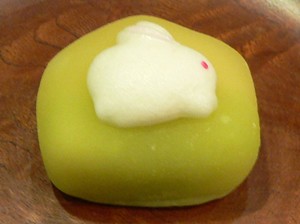This image depicts a light green bar of soap sitting on a variegated wooden table with a medium to dark brown finish. The table's wood grain features lines and a slight glare, and it has an area that's lighter towards the corner. On top of the soap is an irregularly shaped mass of white soap suds, with a very small red dot on the right side of the suds. The item is centrally placed on the table, casting a shadow in the foreground that suggests the light source is from directly behind at an angle. There's nothing else in the image to provide additional context.